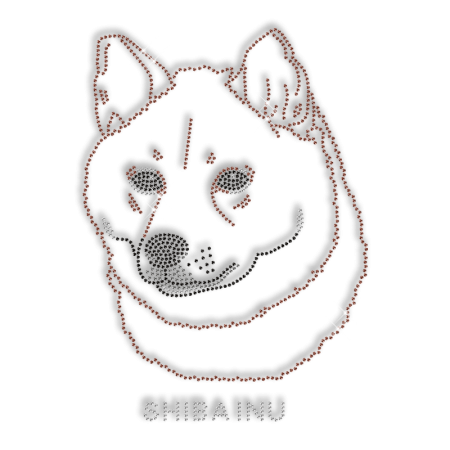This image features a stylized, dotted portrait of a Shiba Inu, meticulously crafted using a series of dots to form its distinct features. The dog is primarily depicted in shades of dark tan and black, with the brownish-tan dots outlining its ears, neck, and face. Black dots are used to intricately define its eyes, nose, mouth, and whiskers, highlighting the dog's expressive features. The Shiba Inu appears primarily white with detailed dot work emphasizing its contours. Below the dog, the label "Shiba Inu" is spelled out in gray dots, accompanied by a solid, light-gray shadow that adds depth to the text and subtly appears throughout the image. The image, reminiscent of the famous Dogecoin Shiba Inu, utilizes a monochromatic color scheme with hints of a dark reddish-gray, giving it a unique and artistic pixelated look suggestive of a meme style.